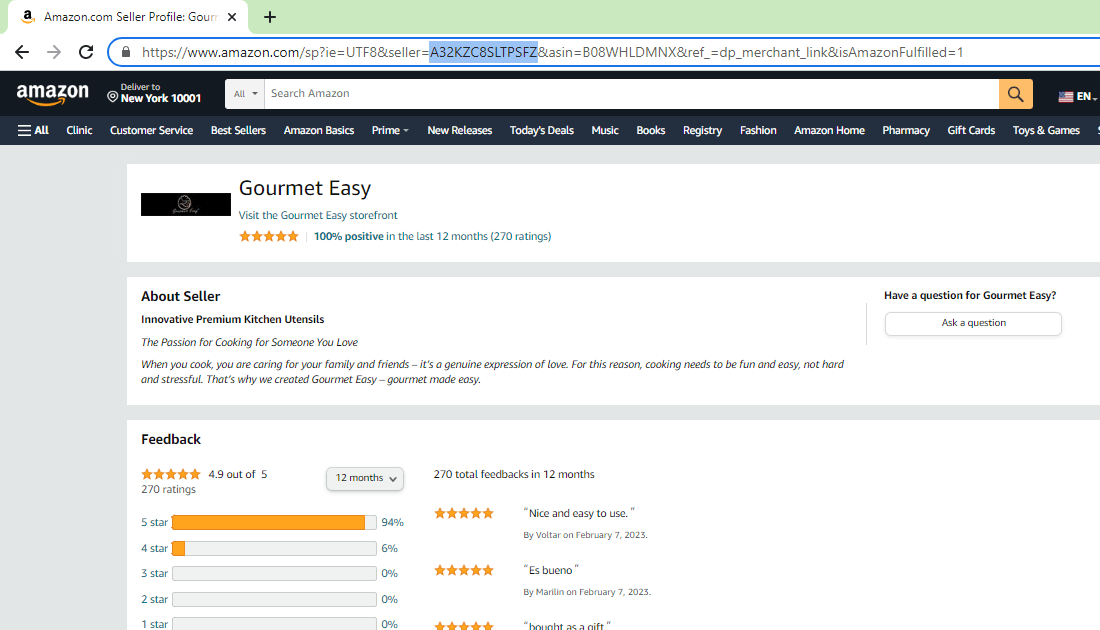This image is a detailed screenshot of a seller's profile page on Amazon.com. At the very top, there is a navigation bar with a green background and an open tab labeled "amazon.com seller profile". The URL in the search bar confirms this is an Amazon.com page.

Directly beneath, there is the standard Amazon.com toolbar, including a search bar and a menu with numerous categories such as All, Clinic, Customer Service, Bestsellers, Amazon Basics, Prime, New Releases, Today's Deals, Music, Books, Registry, Fashion, Amazon Home, Pharmacy, Gift Cards, Toys, and Games.

The background of the page transitions to gray, highlighting several white boxes with information. The first box introduces "Gourmet Easy" with a bold black heading. It states "Visit the Gourmet Easy Storefront" and highlights that the seller has a 5-star rating with 100% positive feedback over the last 12 months from 270 ratings.

Beneath that is an "About Seller" section which describes the seller's dedication to creating innovative, premium kitchen utensils. The description emphasizes that cooking should be an enjoyable and stress-free activity, rooted in a genuine expression of love for family and friends. This philosophy fuels the creation of Gourmet Easy products.

On the right-hand side, there’s an interactive section with the heading "Have a question for Gourmet Easy?", accompanied by a button to ask a question.

At the bottom of the page is a feedback box summarizing the seller's ratings: an impressive 4.9 out of 5 stars from 270 total feedbacks received over the last 12 months, with 94% of the ratings being 5 stars and 6% being 4 stars.